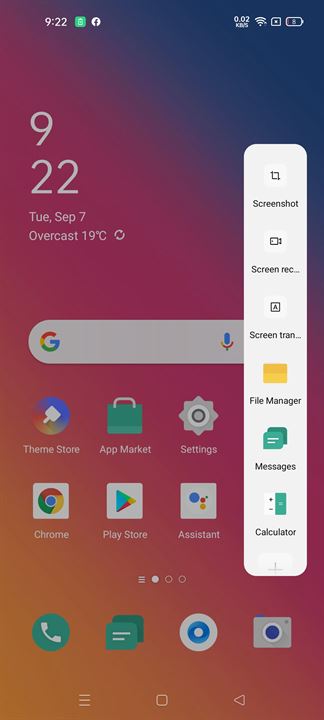The image is a screenshot of a smartphone's home screen, featuring a vibrant gradient background that transitions from dark blue at the top right to pink and finally to orange at the bottom left. On the top left corner, the time is displayed as 9:22, accompanied by a green icon and the Facebook icon. The top right corner houses the signal strength indicator and the battery life icon.

Below the time, centrally aligned but not at the very top, the date and weather details are displayed: "Tuesday, September 7th, overcast, 19°C", along with an option to refresh. There is a vertical pop-up on the screen enclosed in a white rectangle, featuring various menu options including: Screenshot, Screen Record, Screen Transfer, File Manager, Messages, and Calculator.

In the center of the screen, a Google search bar is prominently featured. Scattered across the background are several app icons: Theme Store, App Marketplace, Settings, Chrome, Play Store, and Assistant. This is the primary home screen of three available, indicated by the screen indicator at the bottom; swiping to the right will reveal a different screen.

At the bottom of the screen, just above the screen indicator, are four icons: Phone, Messages, Internet, and Camera. Below these, there is a menu bar featuring three navigational icons: a circle for Home, a square for Recent Apps, and a backwards triangle for Back.